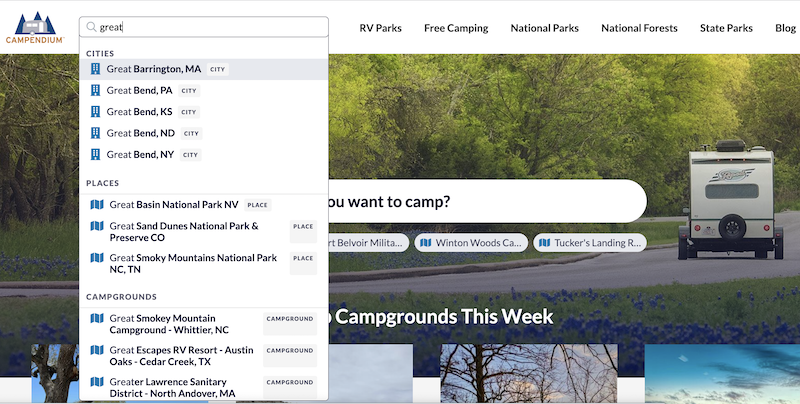This image is a detailed screenshot taken from a web page in landscape mode. In the upper left-hand corner, a logo reads "Campendium." To its right, a search bar contains the text "G-R-E-A-T," with the cursor positioned at the end of the word, prompting a drop-down menu. The menu lists several search suggestions spanning different categories: 

**Cities:**
- Great Barrington, Massachusetts
- Great Bend, Pennsylvania
- Great Bend, Kansas
- Great Bend, North Dakota
- Great Bend, New York

**Places:**
- Great Basin National Park, Nevada
- Great Sand Dunes National Park and Preserve, Colorado
- Great Smoky Mountains National Park, North Carolina and Tennessee

**Campgrounds:**
- Great Smoky Mountain Campground, Whittier, North Carolina
- Great Escapes RV Resort, Austin, Oaks, Cedar Creek, Texas
- Greater Lawrence Sanitary District, North Andover, Massachusetts

Just below the search bar and drop-down menu, the top row of the web page features navigation headers: RV Parks, Free Camping, National Parks, National Forests, State Parks, and Blog. Below this navigation bar, a large background image predominantly shows a lush, green landscape. The image features a road that begins on the left side and extends diagonally upward to the right, where a small camper is visible near the center-right.

Central to the page, another search bar is displayed with the prompt "You want to camp?" Below this prompt, several buttons are labeled with campsite names: Belvoir Military, Winton Woods, CA, and Tucker's Landing. Beneath these buttons, a section titled "Campgrounds this week" is visible. The webpage is only partially scrolled, revealing upper portions of the images and content further down.